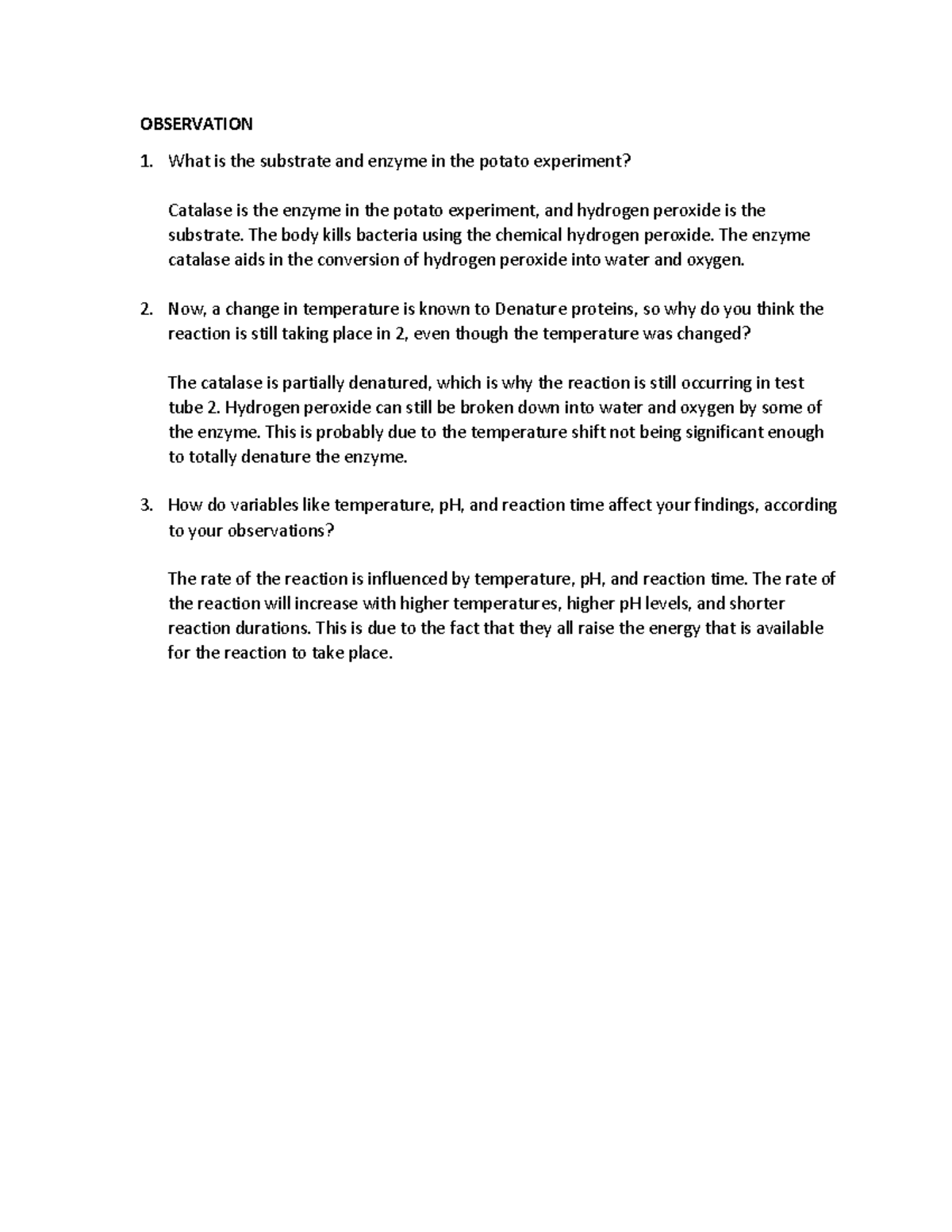**OBSERVATION**

1. **What is the substrate and enzyme in the potato experiment?**

   In the potato experiment, catalase is the enzyme, and hydrogen peroxide is the substrate. The body utilizes hydrogen peroxide to kill bacteria. Catalase aids in the conversion of hydrogen peroxide into water and oxygen.

2. **A change in temperature is known to denature proteins. Why do you think the reaction is still taking place in Test Tube 2, even though the temperature was changed?**

   In Test Tube 2, the catalase enzyme is only partially denatured, which is why the reaction is still occurring. Hydrogen peroxide can still be broken down into water and oxygen by some of the enzyme. This is probably because the temperature shift was not significant enough to completely denature the enzyme.

3. **How do variables like temperature, pH, and reaction time affect your findings according to your observation?**

   Temperature, pH, and reaction time all influence the rate of the reaction. Higher temperatures, higher pH levels, and shorter reaction durations increase the rate of reaction. This is because they all raise the amount of energy available for the reaction to take place.